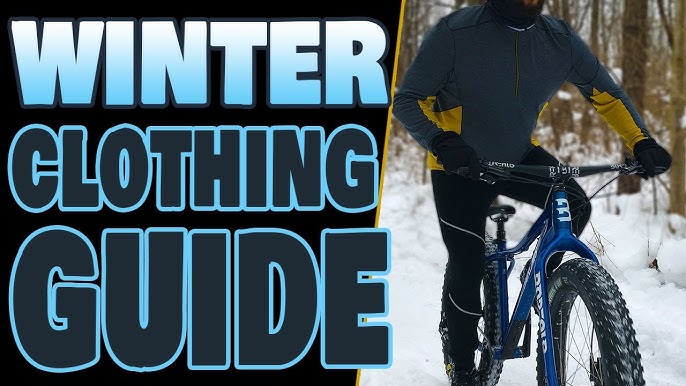This image is a promotional poster for a winter clothing guide. The left side features large text reading "Winter Clothing Guide" with the word "Winter" in a gradient from light blue to white and "Clothing Guide" in dark grey, all set against a solid black background. This text takes up a little over half of the visible space. A gold line separates the text from the right side of the poster, which displays a photograph of a man riding a blue and black mountain bike through a snowy forest. Only the man's torso and part of the bicycle are visible as his head is cut off in the image. He is dressed in winter attire, including a grey and yellow jacket, black pants, and black gloves. The scene is framed by snow-covered ground and the trunks of bare trees, emphasizing the winter environment.